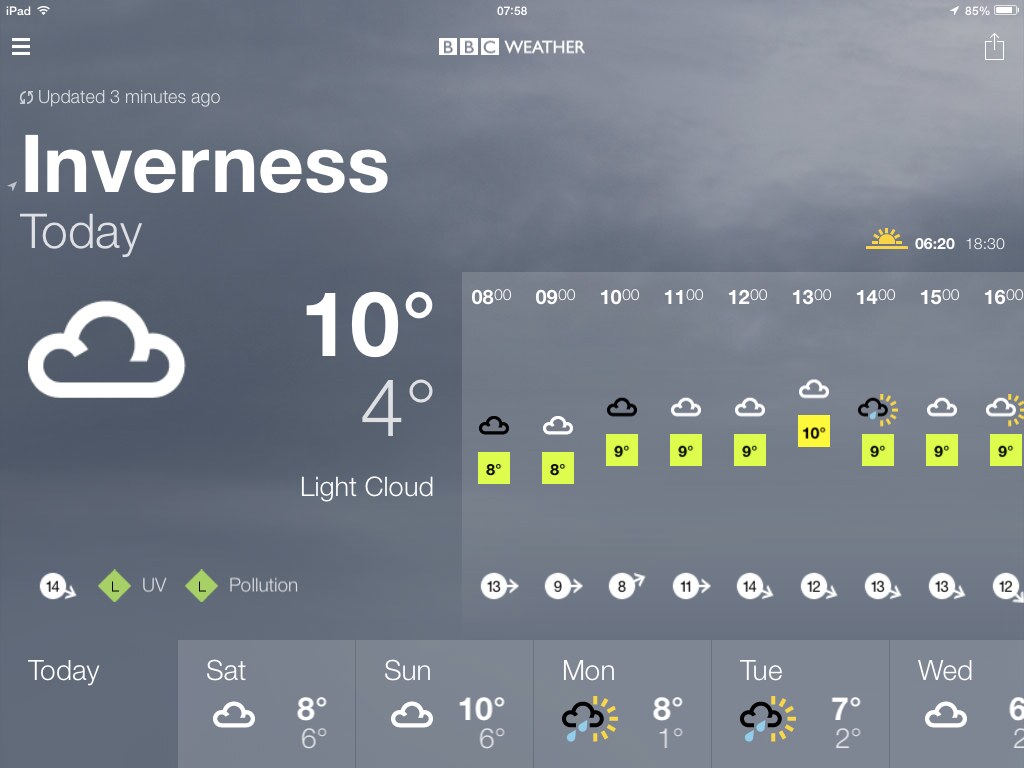This image is a color screenshot in landscape orientation, displaying a weather forecast from the BBC Weather website, captured on an iPad, as indicated by the white text "iPad" in the upper left corner, along with the Wi-Fi signal, the time "7:58," and an 86% battery indicator in the upper right. The main section of the screenshot features a light cloud background with a large white text "Inverness" and a subheading "today." A bold white cloud icon is centered below this text, with temperatures prominently shown as "10 degrees" and "4 degrees Celsius" underneath, alongside a description "light cloud." A vertical hourly chart spans across the screen, detailing the weather from 8 o'clock through to 16 o'clock with corresponding icons. Towards the bottom left, a brief forecast indicates low pollution and UV levels, while an extended outlook covers Saturday through Wednesday, showing varying weather conditions from cloudiness to sun showers and their corresponding temperature ranges.